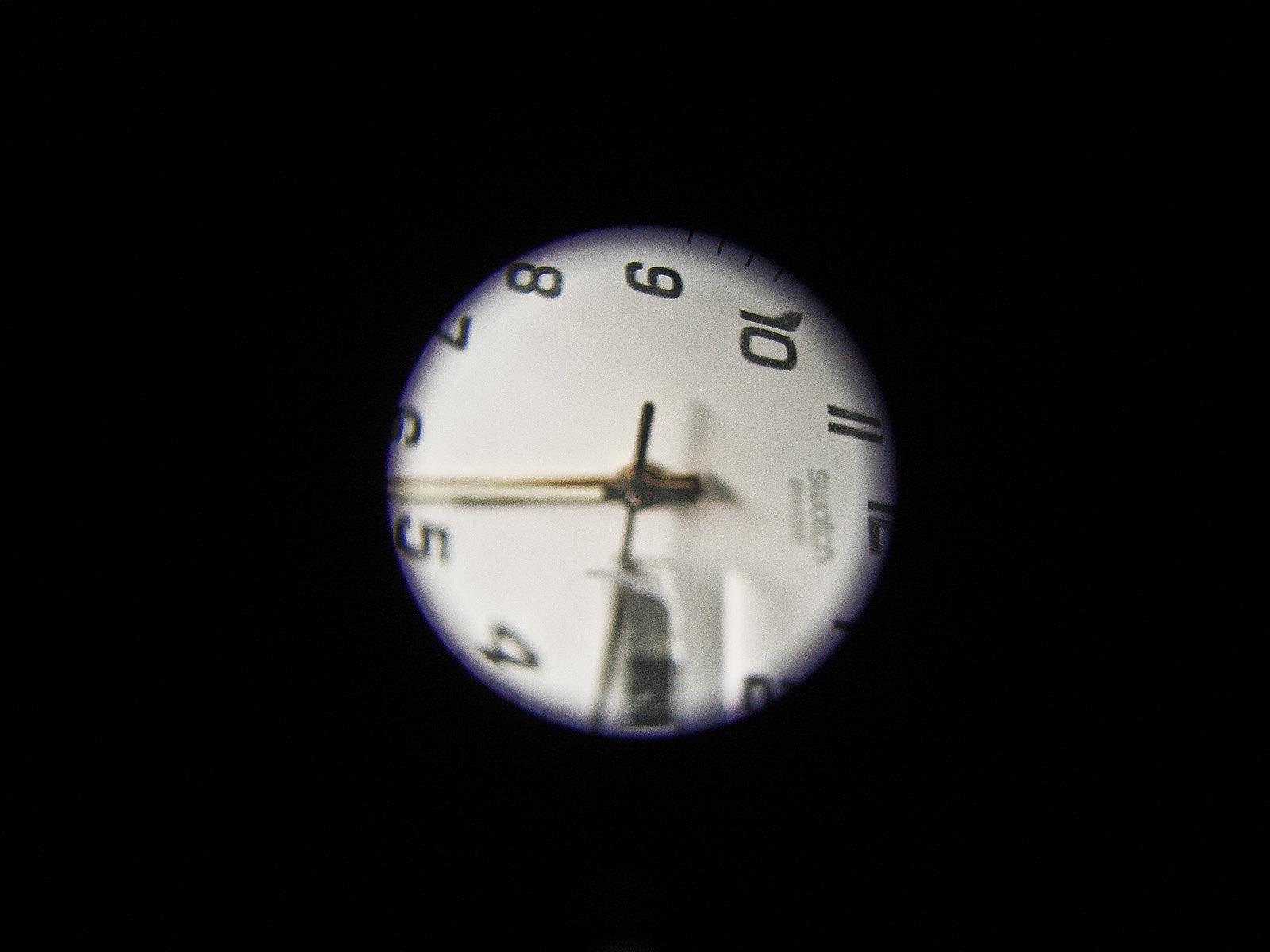The photograph is a contemporary piece, predominantly enveloped in black. At the heart of the image lies a nearly perfect circle, which appears to be the face of a wristwatch. The transition from the stark black surrounding to the white central circle is gently faded, creating a subtle gray gradient at the junction rather than a harsh dividing line.

Upon closer inspection, the watch face reveals its markings. The numerals 8, 9, 10, 11, 4, and 5 are fully visible, while the numbers 7, 6, 12, 1, 2, and 3 are only partially seen, yet discernible. Positioned just beneath the 12 is the brand name "Swatch," indicating the watch's manufacturer.

In the center, the minute and hour hands are prominently displayed, with no second hand present. Adjacent to the 3 o’clock mark, a small window is visible, likely intended for the date display. Notably, the entire watch face is oriented sideways within the frame, adding an intriguing angle to the composition.